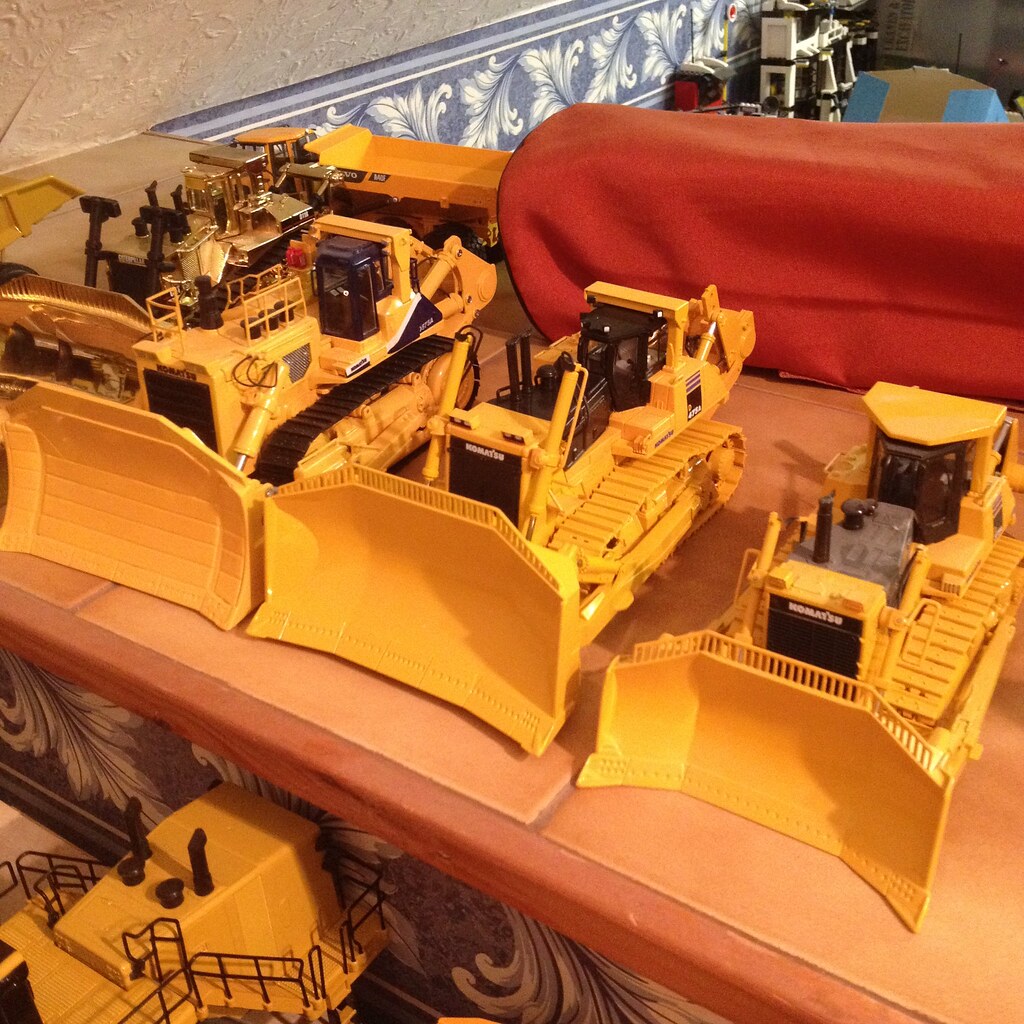The photograph depicts a detailed indoor scene featuring three large, realistic-looking yellow toy bulldozers arranged side by side. These toy bulldozers, sporting the brand name 'Komatsu' on a black panel with white text, are primarily yellow with black accents, including black cabins and black tops on the engines. They are set on a pink salmon-colored table that appears to have large beige tiles as its surface. In the background, a blue and white lining, possibly floral wallpaper, is visible along with some additional objects including another yellow tractor toy, a red cloth cover, and a yellow dump truck. The image, in a square format, provides a vivid and intricate depiction of a miniature construction scene.